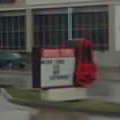In this image, a small thumbnail-sized photo, the marquee board of an Arby's restaurant is prominently displayed in the foreground. The Arby's logo is positioned on the right side of the marquee board, which features a white background bordered by a red strip at the top with the words "drive-thru" written in white letters. The black text on the white area of the board is difficult to discern due to the image's size. The marquee is mounted on a rectangular pedestal, giving it a three-dimensional appearance. Behind the marquee, a building with large windows can be seen, likely a commercial retail space. The ground around the sign appears to be wet, suggesting recent rainfall.